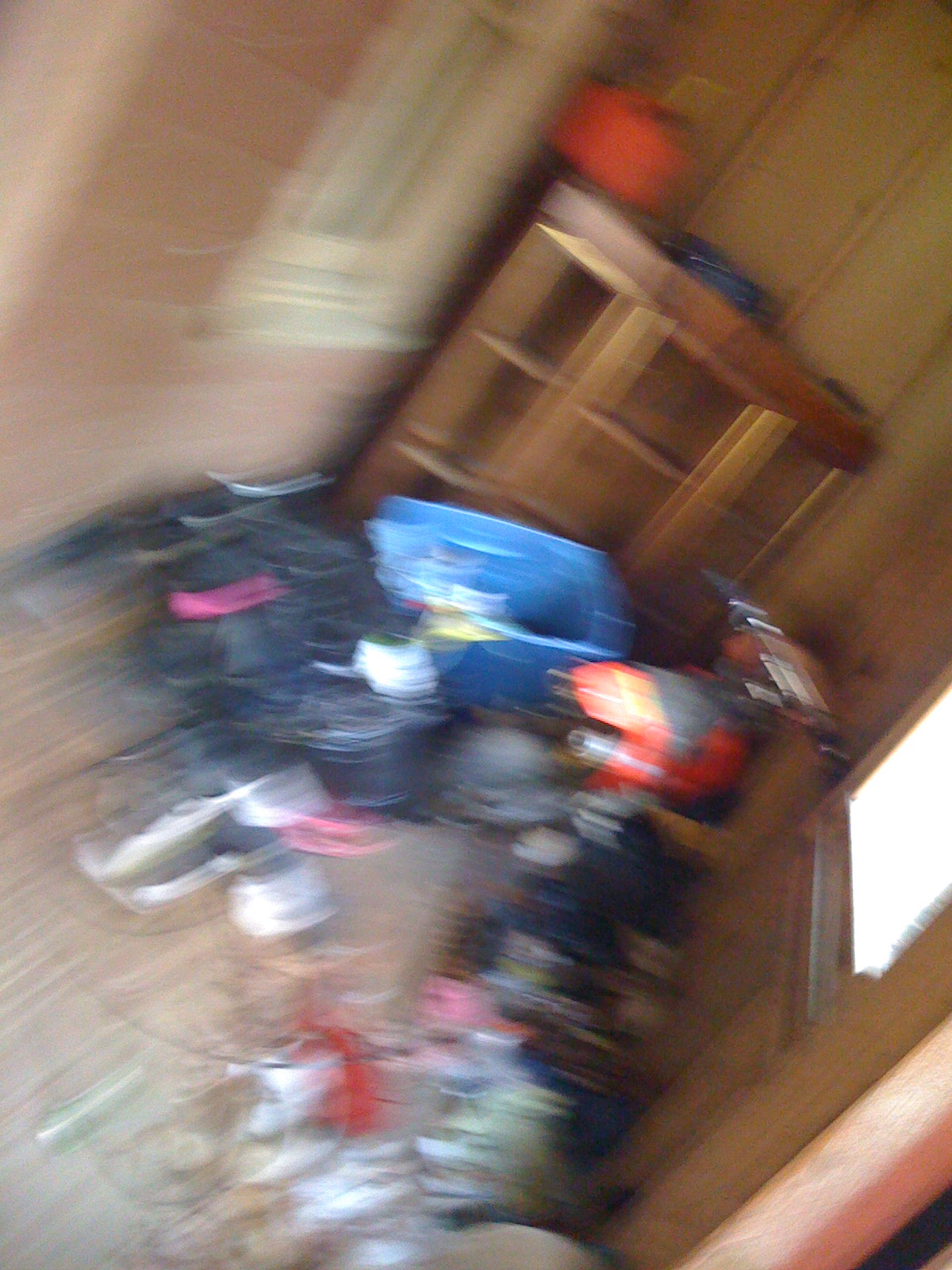This blurry and out-of-focus photograph captures a chaotic corner of a room, where two walls with differing textures and colors meet. The left wall appears to be painted a pink hue and features a window with a white frame that allows some light to filter through. The right wall is made of natural wood paneling. 

In the corner, there's a piece of wooden furniture, possibly a cabinet or shelf, with an orange object resting on top of it. In front of this furniture, a large blue tub stands surrounded by a heap of clothes or garbage scattered across the wooden floor. 

To the right of the tub, partially obscured by the chaotic scene, is a motorbike with a reddish base, its front tire pressed against the wall, and its back tire pointed outward. Overall, the scene is extremely messy, with indistinguishable items contributing to the overall clutter.